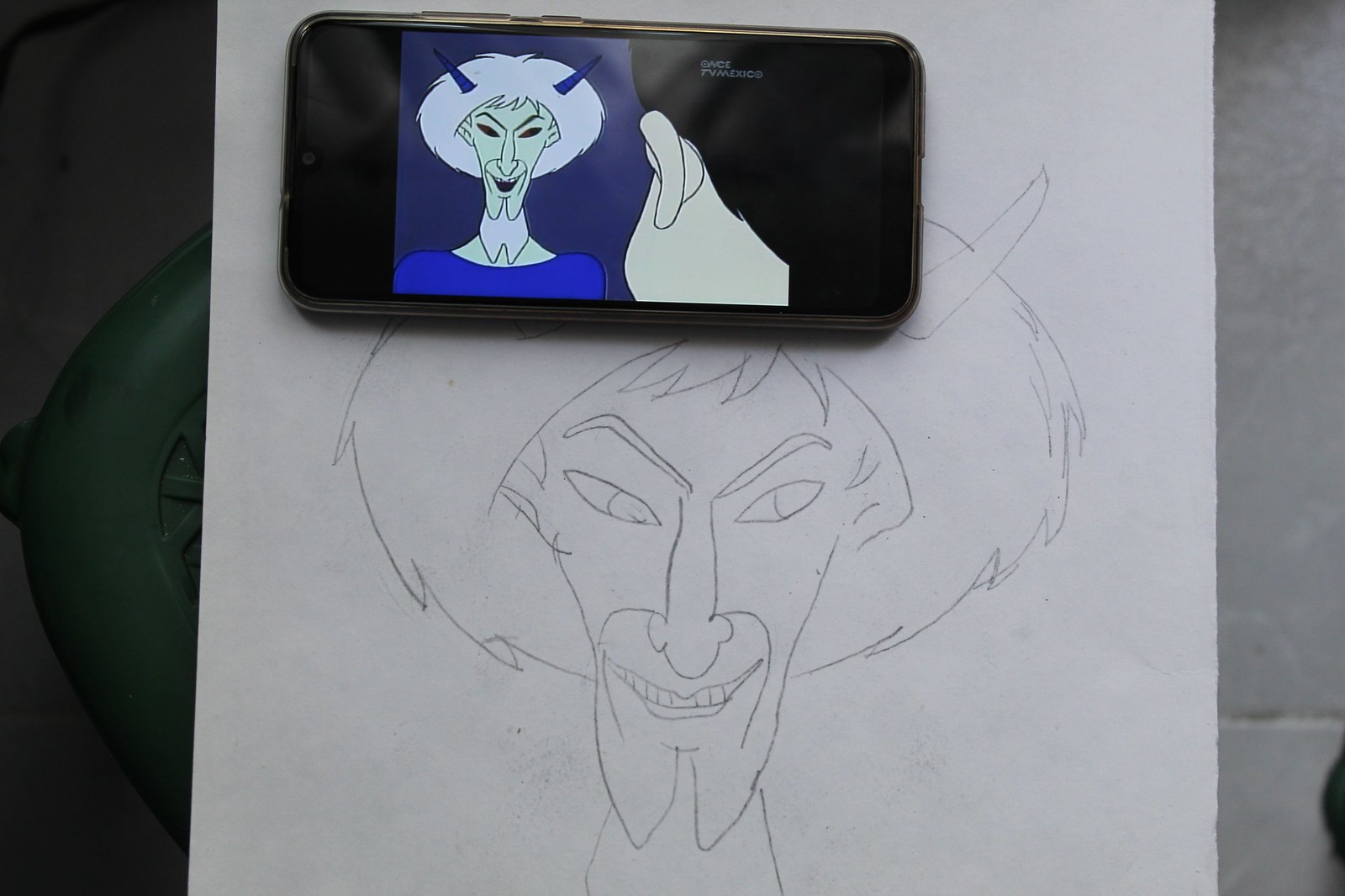The color photograph captures a detailed and precise pencil sketch of a devilish character on a piece of white paper, centered in the frame. The sketch, which is only of the character's head, depicts the figure with fluffy white hair, blue horns, slanted red eyes beneath angled eyebrows, a large nose, and a distinctive goatee, resembling a cow hoof. Just above the sketch and covering part of it, a black smartphone is placed horizontally. The phone’s screen displays a reference image, likely a screenshot from an anime or cartoon, of the same devilish character. In the reference image, the character wears a bright blue shirt and is accompanied by the back of a little girl with black hair, visible to the right. Although there's white text on the girl's head in the reference image, it's too small to be legible. The smartphone and paper share the same landscape orientation, highlighting the artist's impressive skill in replicating the character's likeness from the screen to the sketch. The accuracy of the illustration underscores the artist’s talent in capturing the character’s sinister expression and detailed features.